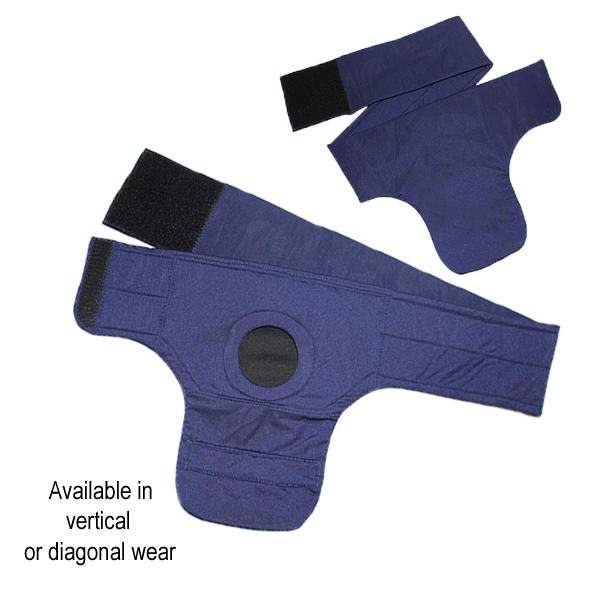The image is a detailed advertisement of a blue and black cloth product designed with adjustable Velcro straps, featuring two views of the item. Primarily blue, the object has a distinctive hole in its middle, possibly to accommodate a tail or some sort of protrusion, suggesting it could be a specialized item, perhaps a diaper for pets. The main view in the center showcases the front side of this uniquely crafted gear, while a smaller inset to the top right displays the back side, which lacks the hole seen in the front. Both views highlight the blue material and the securing black Velcro ends. The product's versatility is emphasized by the black text in the lower left corner, stating "available in vertical or diagonal wear," hinting at its multi-functional design.